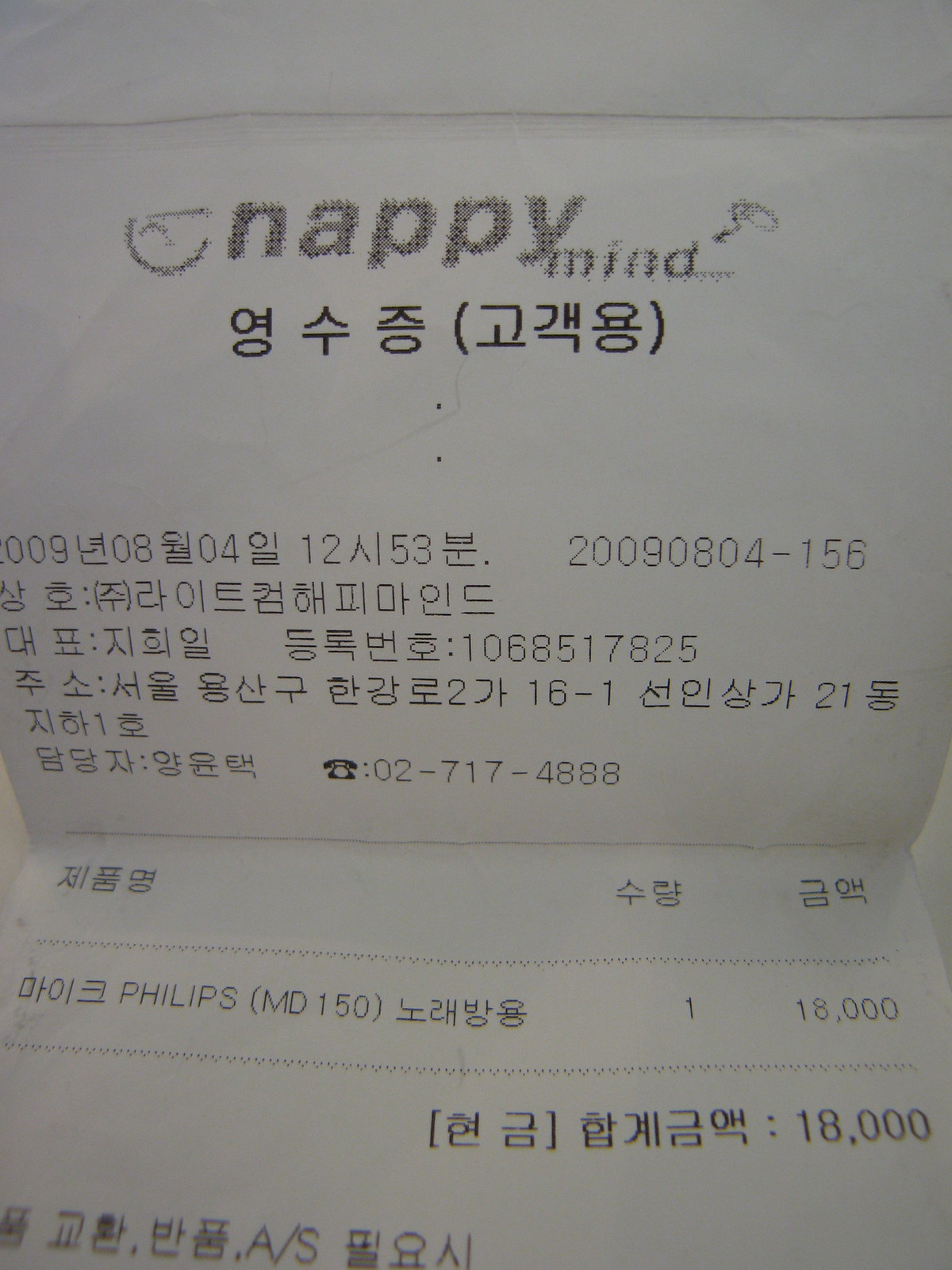The image depicts a receipt from a South Korean store named "Nappy Mind." The receipt is primarily printed in Korean, with the store's name and the product details in English. A Philips MD-150 was purchased for 18,000 Korean Won. The receipt includes additional details such as the store's telephone number, which is 02-717-4888, and other relevant information mainly in Korean characters.